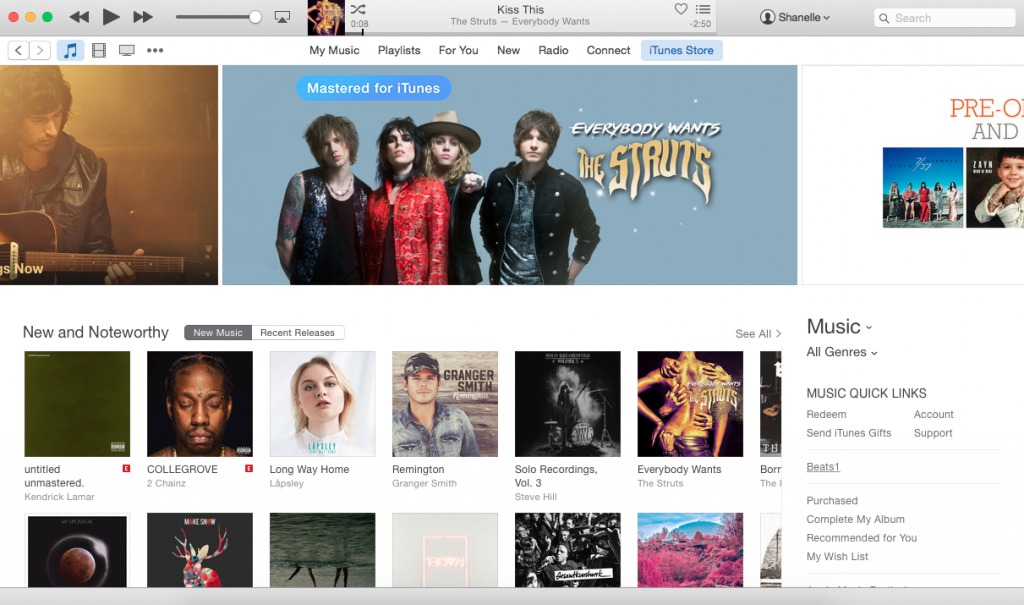The image depicts the interface of a music website that strongly resembles iTunes, known for its dated aesthetic. At the top of the interface is the iconic, unchanged iTunes bar. Directly below this is the main menu, featuring tabs such as 'My Music,' 'Playlist,' 'For You,' 'New,' 'Radio,' and 'Connect.' 

The primary section of the page has a clean white background adorned with various pictures and text in black. A sidebar on the left provides easy navigation links to different music categories, including 'All Genres,' 'Music,' 'Quick Links,' and 'Beats.'

At the very top of the central content area, prominent featured images highlight selected content. The only fully visible featured image displays a promotional banner with the text "Everyone Wants the Struts," showing the band posing against a gray background. Below this banner, a section titled 'New and Noteworthy' presents a collection of album covers arranged neatly in rows and columns, showcasing the latest music releases.